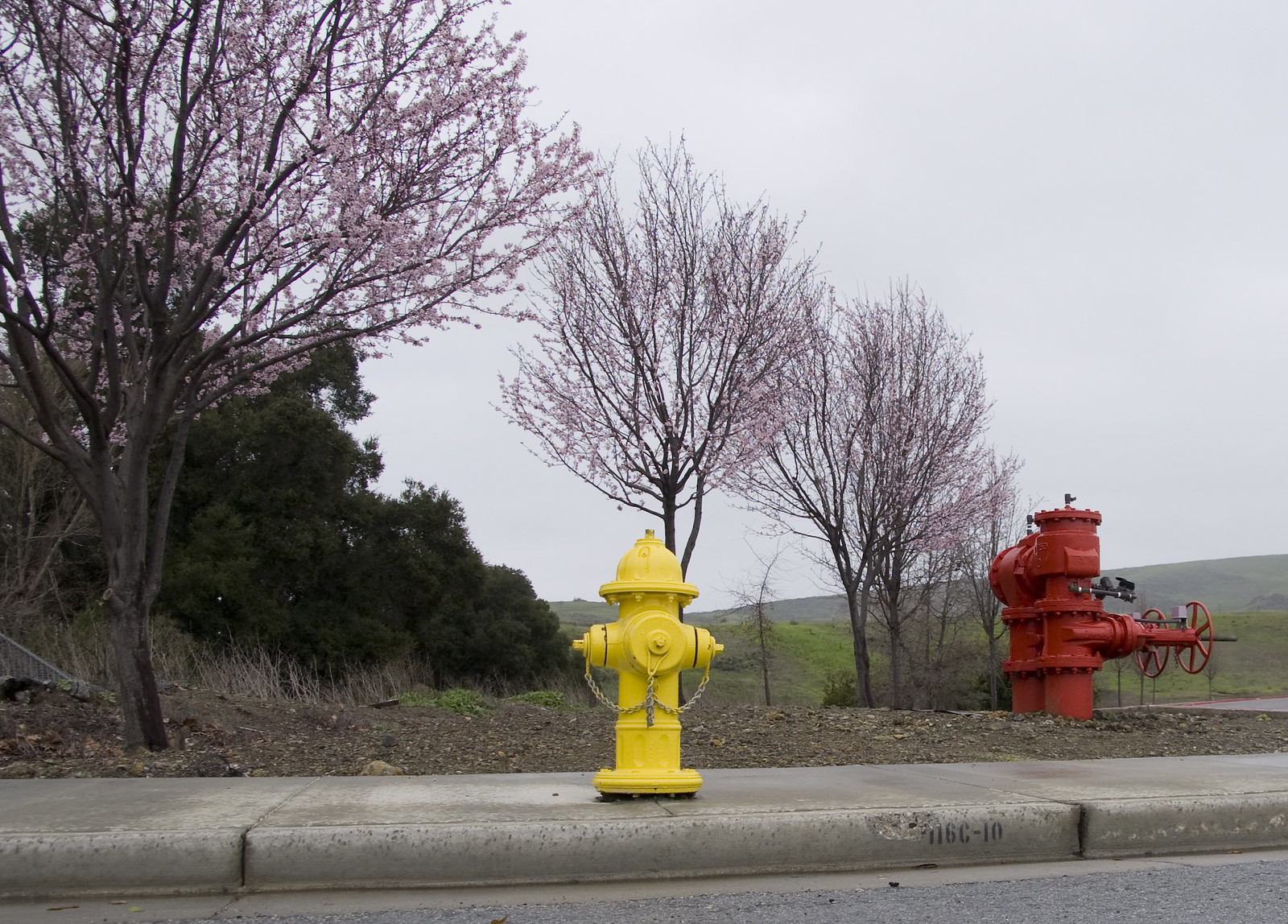The photograph captures an outdoor scene taken from a low angle near street level, focusing on a bright yellow fire hydrant positioned centrally on a curbside sidewalk. The hydrant appears freshly painted with attached yellow chains. To the right of the hydrant stands a larger, industrial-looking red pipeline assembly, featuring two prominent valves, likely used for water management. This red valve assembly is considerably larger than the fire hydrant, extending about two meters high.

The foreground includes a portion of the roadway and the sidewalk, which has "116C-10" written on it. The midground consists of a patchy area with brown gravel, some sparse grass, and mulch. Several thin, leafless trees and green bushes populate this area, suggesting a late autumn or early winter setting. Off to the left in the background, evergreen trees and lush shrubbery can be seen, while the right side features a gradually inclining hill.

The backdrop of the photograph is dominated by an overcast, gray sky, giving the scene a melancholic and rainy day atmosphere. Further in the distance, the image captures a horizon line featuring hills or possibly mountains with a misty appearance, enhancing the overall moody ambience of the scene.